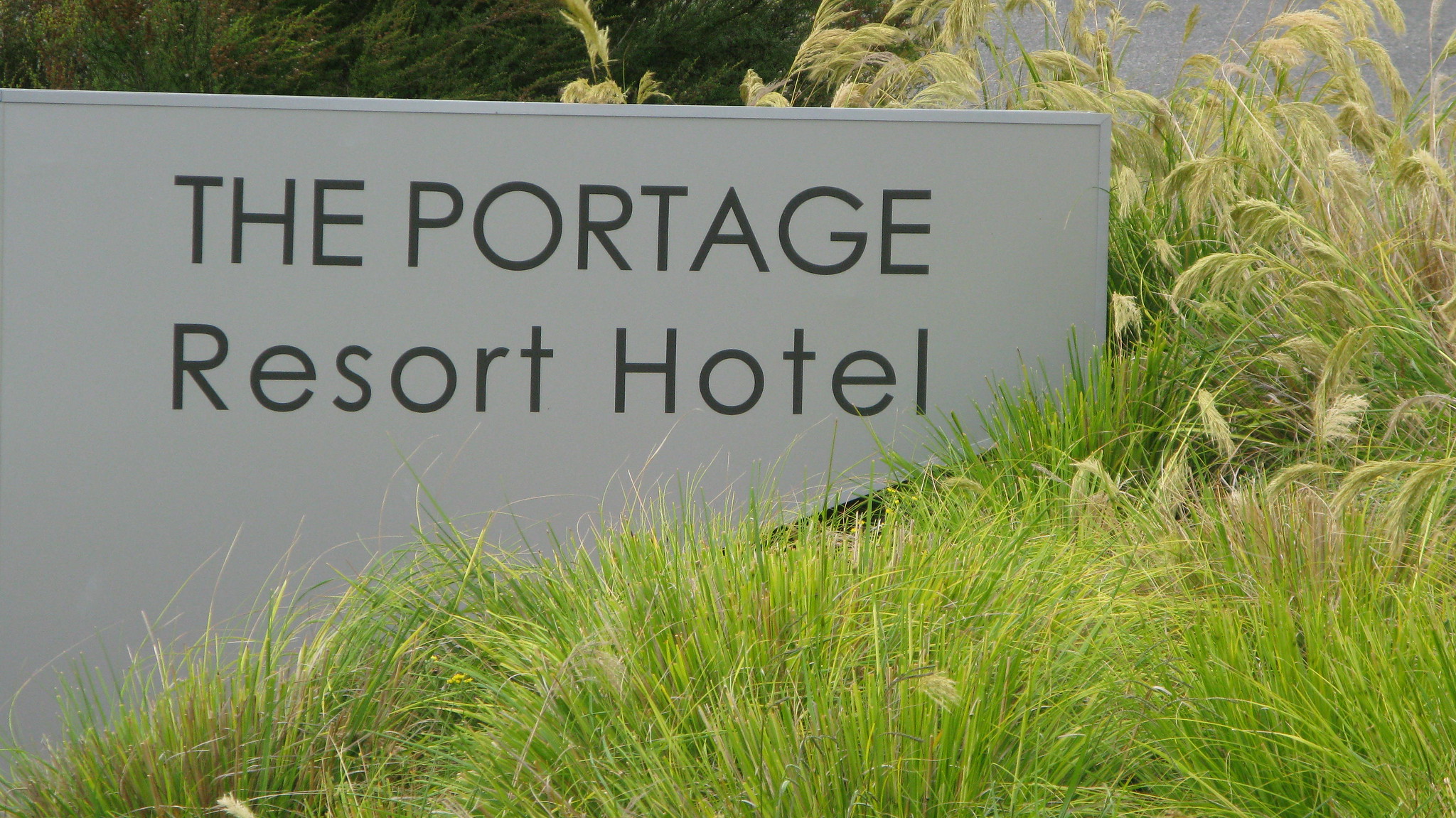The image showcases an outdoor sign for "The Portage Resort Hotel." The sign's off-white base supports large, dark gray capital letters that read "The Portage," with smaller capitalized letters spelling out "Resort Hotel" beneath. It is prominently clean and displays a sleek, smooth appearance. The backdrop and surroundings are lush with various types of long grasses and wild vegetation. To the right of the sign, tan-colored, straight-leaved weeds dominate the scene, spilling over and obscuring the area. The background features darker green foliage, possibly trees or dense bushes, adding depth to the landscape. The sign appears slightly angled, with much of its right side enveloped by plant life, enhancing its integration with nature. It stands alone without visible support structures, suggesting a seamlessly blended natural setting, potentially marking an entrance to the resort.